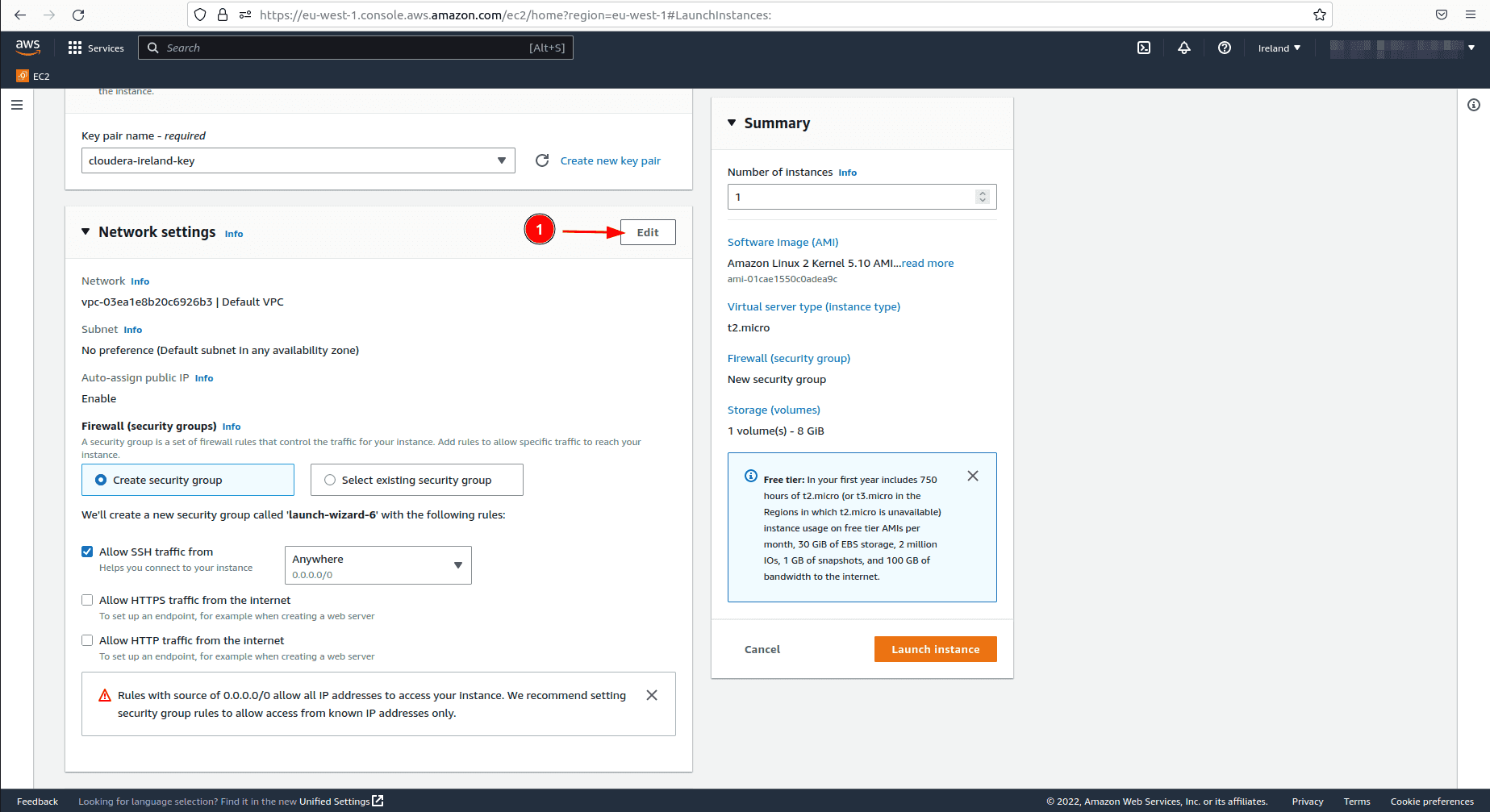Screenshot of Amazon Web Services (AWS) Management Console in the Ireland region, showcasing the setup process for launching an EC2 instance:

The console displays various configuration sections that an administrator might encounter. Key details include:

1. **Key Pair Configuration**: Named "CloudAero-Ireland-key".
2. **Network Settings**: Configured to use a specific Virtual Private Cloud (VPC) with a subnet preference set to "No preference". The option "Auto-assign Public IP" is enabled.
3. **Security Group Settings**:
    - A new security group named "Launch Wizard 6" will be created.
    - The only enabled rule permits SSH traffic from any IP address, enhancing secure server access.

Highlighted in the image, a red arrow and red circle emphasize the "Edit" button under the network settings, providing clarity on where adjustments can be made.

Summary details on the right side of the screen include:
- **AMI**: Amazon Linux Kernel 2 software image.
- **Instance Type**: t2.micro.
- **Storage**: One volume of 8 GB.
- **Free Tier Information**: Indicates eligibility for 750 hours of t2.micro or t3.micro instances (where t3 is not available) in the first year.

Overall, the screenshot encapsulates the pre-launch configuration step of an EC2 instance, highlighting free tier eligibility and fundamental setup details.